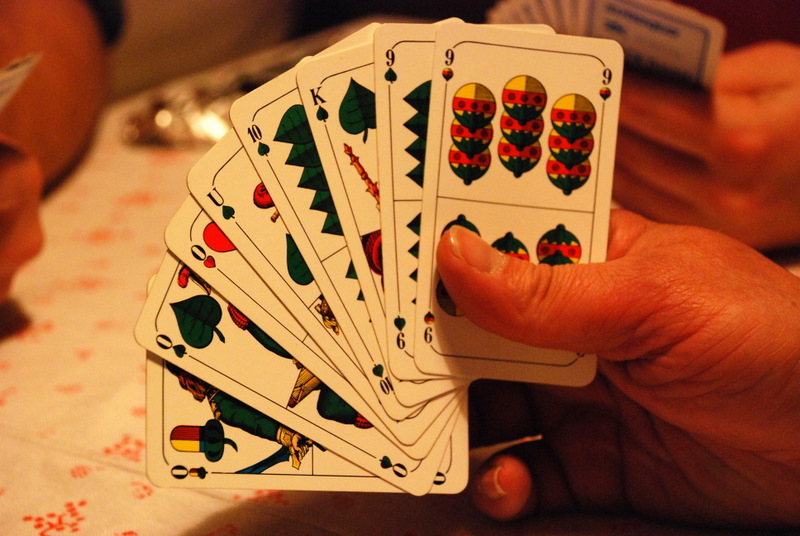The image depicts a close-up view of a table, elegantly covered with a white cloth adorned with delicate red patterns resembling small flowers or leaves. In the foreground, a couple of hands are visible, each holding a hand of unusual playing cards. The cards feature a distinctive design with a light beige background. One card, a nine, is decorated with motifs resembling hot air balloons, each balloon sporting a yellow top, a red middle with three black dots, and a black bottom. Another card, identified as the nine of spades, features black shapes reminiscent of saw blades. The background appears slightly blurred with a soft red hue, adding warmth to the scene. A shiny silver tray rests on the table, contributing to the overall elegant and inviting atmosphere.